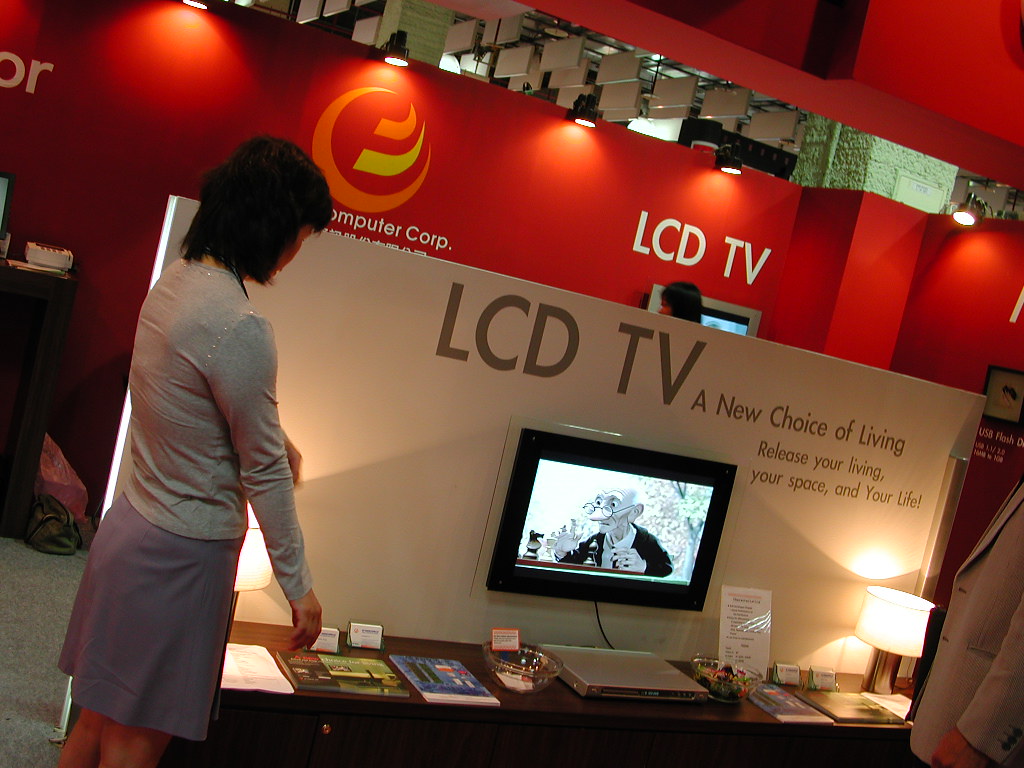The image depicts a modern, trade show booth, possibly at an event like the Consumer Electronics Show (CES). In the background, there is a red, cubist-inspired display adorned with metallic objects hanging from the ceiling. Prominent white text reads "LCD TV, a new choice of living. Release your living, your space, and your life," indicating a promotional focus on innovative living solutions.

A large brown desk occupies the foreground, organized with numerous brochures, pamphlets, and a gray electronic device. A screen with a black border, showing an elderly figure that appears animated or puppet-like, is centrally placed on the desk. Additionally, a flat-screen TV plays a Pixar short, connected via a small cable to a DVD player on the table.

A woman with short black hair, dressed in a light gray long-sleeved blouse and a medium gray skirt, stands to the left, observing the setup. The booth is discreetly lit, featuring two white shaded lamps that add to the modern ambiance. A second figure, clad in a tan blazer, is partly visible at the far right corner, providing a sense of bustling activity within this dynamic trade show environment.